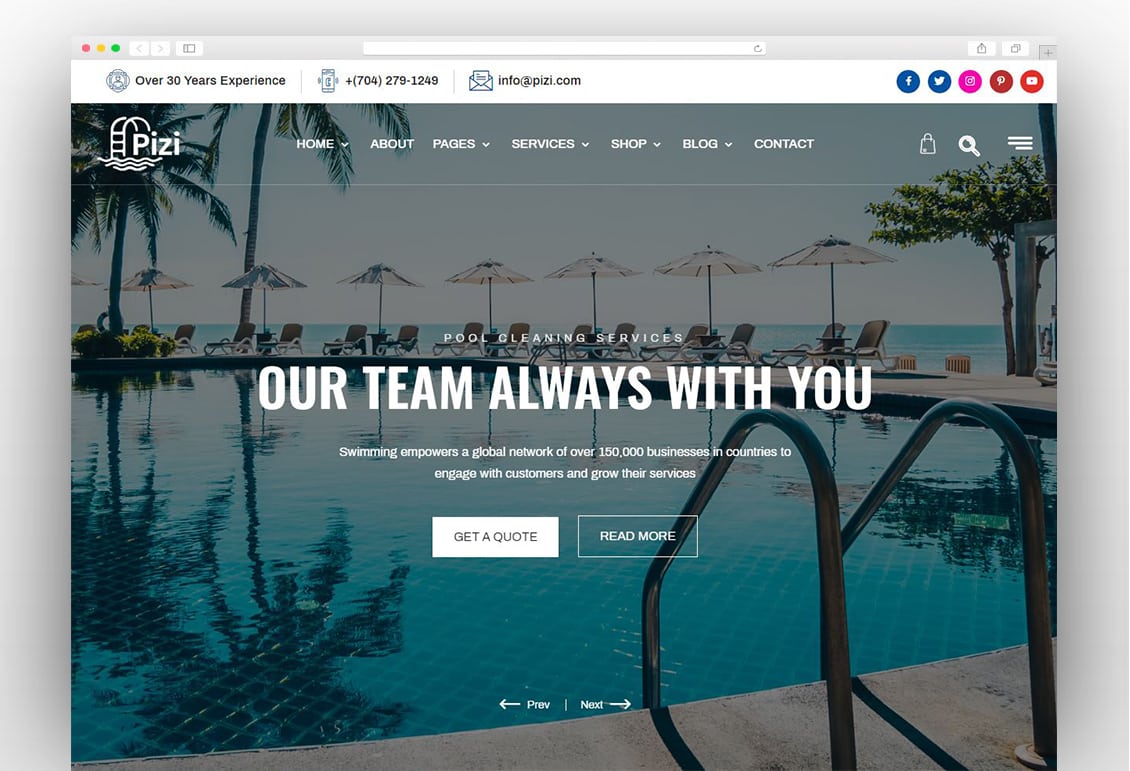A person is browsing a web page on a MacBook, identifiable by the Safari browser. At the top of the web page, there is a white strip featuring an icon resembling a badge, accompanied by the text "Over 30 Years Experience" in black. Below this, an image of a mobile phone is visible, displaying the contact number "(704) 279-1249." Adjacent to this is an email icon with the text "info@PIZI.com."

Towards the right side of the screen, there is a series of circular social media icons. The sequence includes a Facebook icon, a Twitter icon, an indiscernible pink icon, a Pinterest icon, and a YouTube icon.

The main section of the page features a background depicting a pool area with metal handrails on the right, leading into the pool steps. Several umbrellas and a light blue sky can be seen in the background, along with reflections of palm trees in the water.

Centrally displayed in bold, capitalized white letters is the phrase "OUR TEAM IS ALWAYS WITH YOU." Above it, in smaller capitalized white letters with wide spacing, is the text "POOL CLEANING SERVICES." Beneath this, in even smaller print, is the description: "Swimming empowers a global network of over 150,000 businesses and countries to engage with customers and grow their services."

At the bottom, there are two rectangular buttons. The first button has a white background with black text that reads "GET A QUOTE." The second button is transparent, outlined in white, with white text that says "READ MORE."